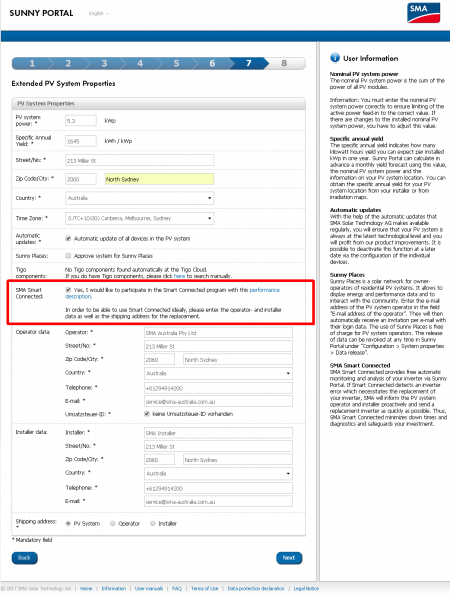This screenshot depicts a web page with detailed structured information and user options. At the very top, the title "Sunny Portal" is prominently displayed in black text. To the right of the title, there is a credit card icon accompanied by the acronym "SMA" rendered in red, white, and blue. A strikingly long, vertical blue bar runs down the page, adding a visual element to separate content.

Below this, another horizontal bar incorporates light blue, dark blue, and white segments, numbered 1 through 8. This numerical bar is followed by the label "Extended PV System Properties." The section beneath features numerous fields and input boxes designed for user information entry, including a conspicuous large red box labeled "SMA Smart Connected." This section has an active checkbox for opting into the "Smart Connected" program, including a performance description.

Among the information fields presented are those for the operator's details, such as street number, zip code, city, country, telephone number, email address, and an ID. Navigation options are provided at the bottom of the page, with blue buttons labeled "Back" and "Next." To the right-hand side of the screen, a series of paragraphs offer additional information. This section begins with the heading "User Information" in black text, accompanied by a blue circle enclosing an "i" icon, indicating further instructive content.